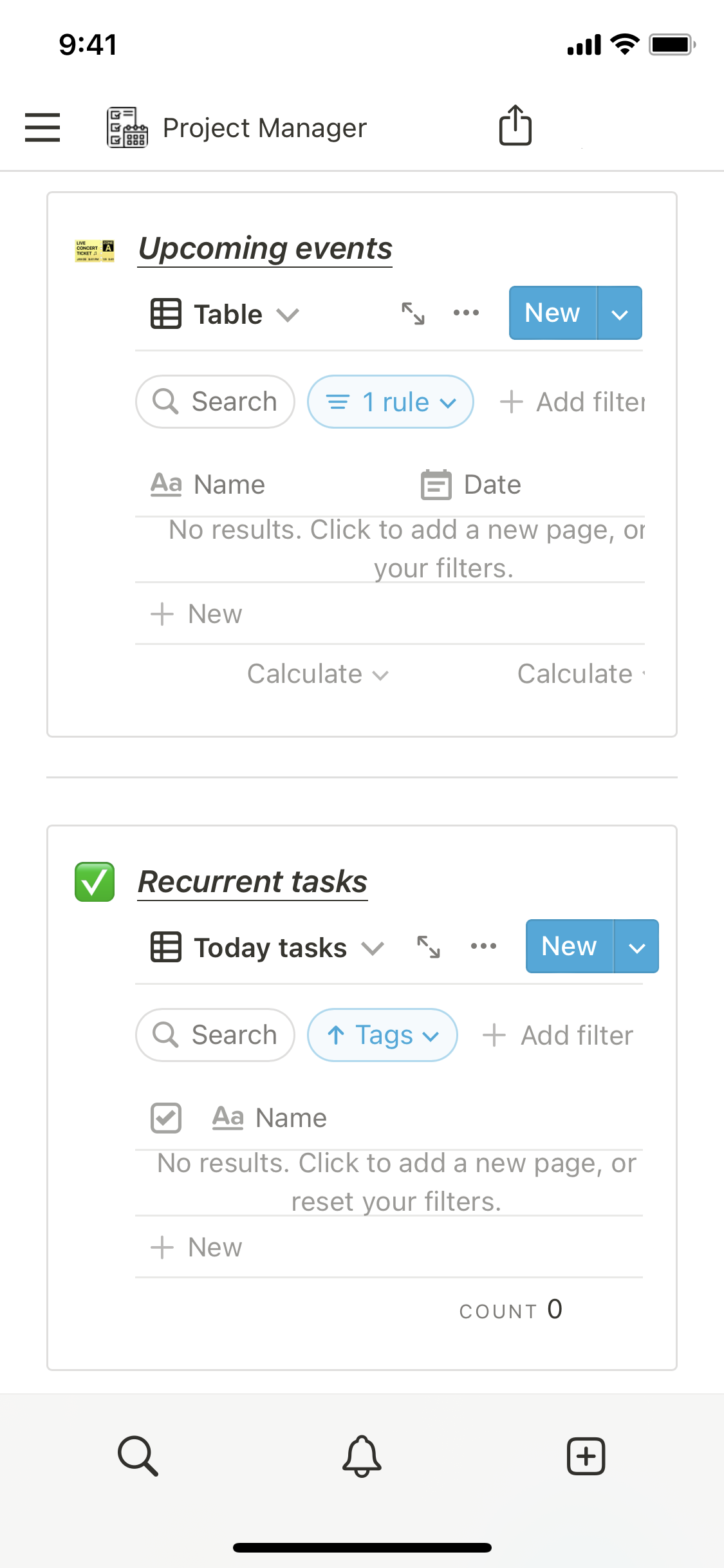The image depicts a cell phone screenshot of a project management application. The interface is streamlined and functional, designed to assist users in organizing their tasks efficiently. The timestamp in the upper left corner reads 9:41, accompanied by icons for signal strength, data strength, and battery level on the upper right. The top section prominently displays "Project Manager," though it remains unclear whether this is a pre-installed app or a third-party download.

The screen is split into two main sections: "Upcoming Events" and "Recurrent Tasks." The "Upcoming Events" section is currently displayed in a table format, suggesting the potential for organizing tasks using various methods such as checklists, critical paths, or dependency charts. Users can also add new tasks, set rules, apply filters, and assign names within this section.

In the "Recurrent Tasks" section, a calendar icon is selected, indicating a focus on scheduling regular activities. This section allows users to add tags, set filters, and perform searches to streamline task management.

At the bottom of the screen, a gray bar houses three essential icons: search, notifications, and a plus icon for adding new items. The notifications icon is underlined, signifying that it is currently active. The overall design of the application highlights usability, making it a versatile tool for organizing tasks and managing time effectively.